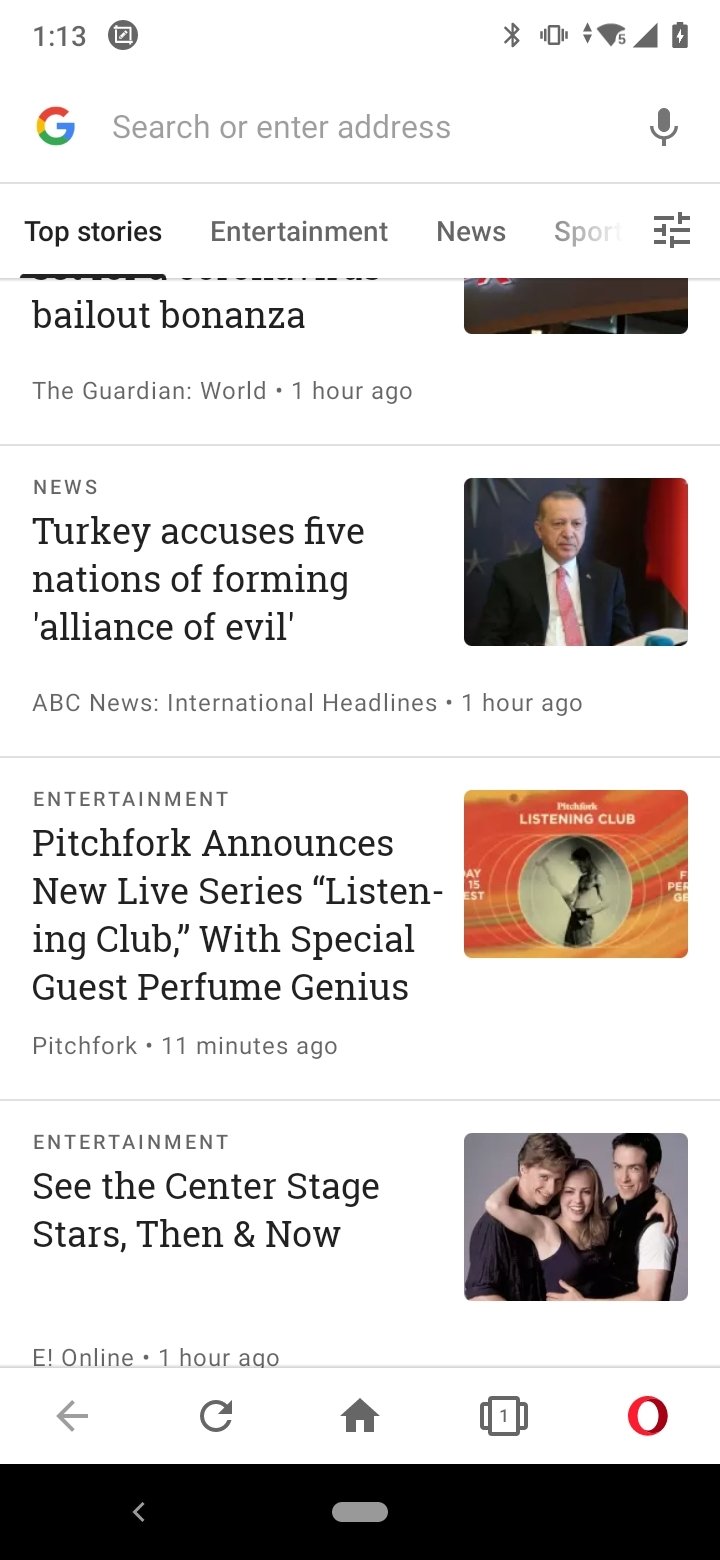The image depicts a smartphone displaying a news app interface. At the top of the screen, there's a search bar labeled "Search or enter address." On the far left, a multicolored "G" icon represents Google, with shades of red, yellow, green, and blue. On the far right, there's a microphone icon for voice searches. Just below the search bar and microphone, navigation tabs categorize the content into "Top Stories," "Entertainment," "News," and "Sports," with an options icon to the right of the tabs. 

Currently, the "Top Stories" tab is selected, indicated by a black underline. The first headline from The Guardian reads "Bailed Out Bonanza," though the title text is slightly obscured; it was published one hour ago. The second headline from ABC News International, titled "Turkey Accused Five Nations of Forming Alliance of Evil," also published one hour ago. The third headline falls under the "Entertainment" category: "Pitchfork Announces New Live Series Listening Club with Special Guest Perfume Genius," from 11 minutes ago. The final headline, also under "Entertainment," is titled "See the Center Stage Stars Then and Now," from E-Online and posted one hour ago. Each headline is accompanied by a small thumbnail image of a person to the right.